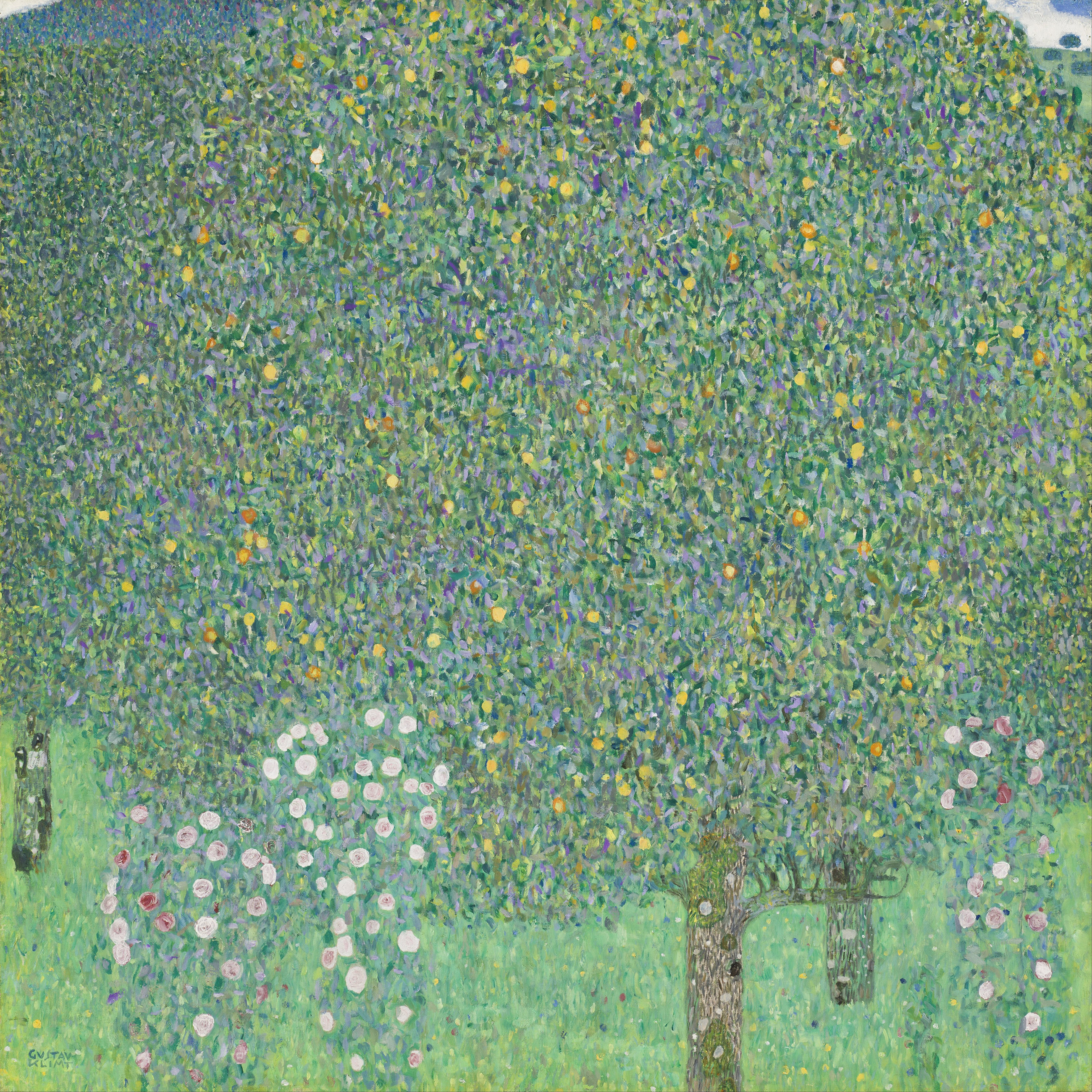This is an impressionistic oil painting by Gustav Klimt titled "Roses Under the Trees," created in 1905. The painting, in portrait orientation, primarily features a large grove of trees dominated by a massive tree in the foreground. The short, straight trunk of this central tree is visible in the bottom right corner and is painted in brown with white spots, extending into a dense, rounded canopy that fills most of the upper portion of the image. The foliage is composed of a stunning array of densely packed dots in pastel hues of green, blue, yellow, and orange, giving it a puffy, almost textured appearance. Among the vibrant leaves, several clusters of orange blossom-like features stand out.

To the left, there’s a cascade of white and pink blossoms, with two smaller tree trunks in the background, adding depth to the scene. The right side similarly features another smaller trunk behind the main tree, with additional white and pink blossoms scattered around. The bottom area of the painting is predominantly green to light green, dotted with tiny specks of other colors, likely representing grass with small flowers. A small section of blue sky with a white cloud is visible in the top right, adding a touch of openness to the otherwise lush depiction. The overall style blends elements of Art Nouveau and modern art, capturing the natural beauty in a vibrant and impressionistic manner.